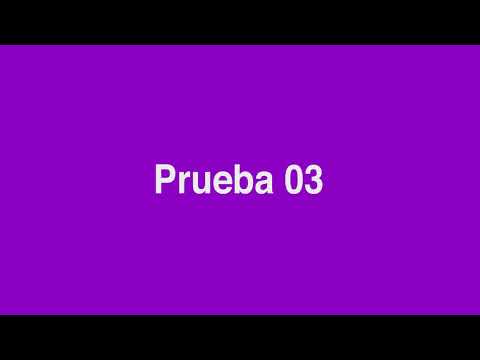The image features a simple, slightly blurry slide or screenshot with a purple background and centered white text that reads "Prueba 03" (Spanish for "Test 03"). There are thin black bars at the top and bottom of the slide, framing the content, but not taking up much space. The text is in a basic sans-serif font, making it easy to read but not overly large. This slide, which may be part of a presentation or projector display, does not include any other text or images, and there are no people visible in the picture.